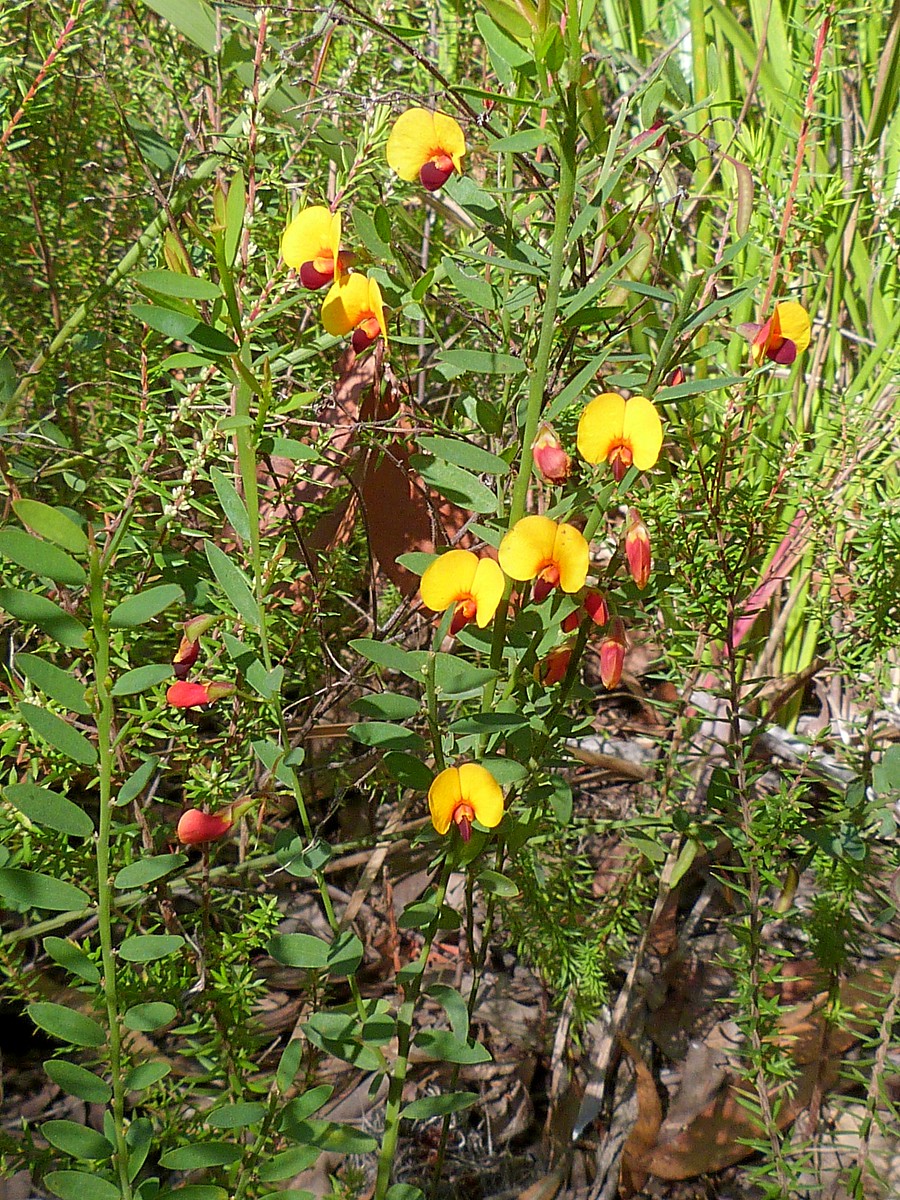The image captures a scene of vibrant wildflowers set amidst a patch of overgrown vegetation. Prominently, there are clusters of moderately tall flowers, approximately a few feet in height, with delicate, yellow petals tinged with subtle red at the centers, resembling the hues of peach slices. Some of these flowers appear unbloomed and display a red, closed form. Surrounding these main flowers, a variety of green plants and shrubs, each with broad leaves growing directly from their stems, create a jumbled tapestry of foliage. Scattered among them are thin, bristled brownish plants with needle-like leaves. The ground is covered in a layer of dried, dead leaves, adding a touch of brown to the scene. Towards the rear of the image, the plants transition to those with long-bladed leaves. The sunlight bathes the entire setting, highlighting the mix of yellow flowers, red buds, green shrubs, and the brown underbrush, suggesting the photo is taken outdoors, likely in a field, garden, or wooded area, during the daytime. This scene exudes a wild, untamed beauty, capturing the essence of nature in full bloom.